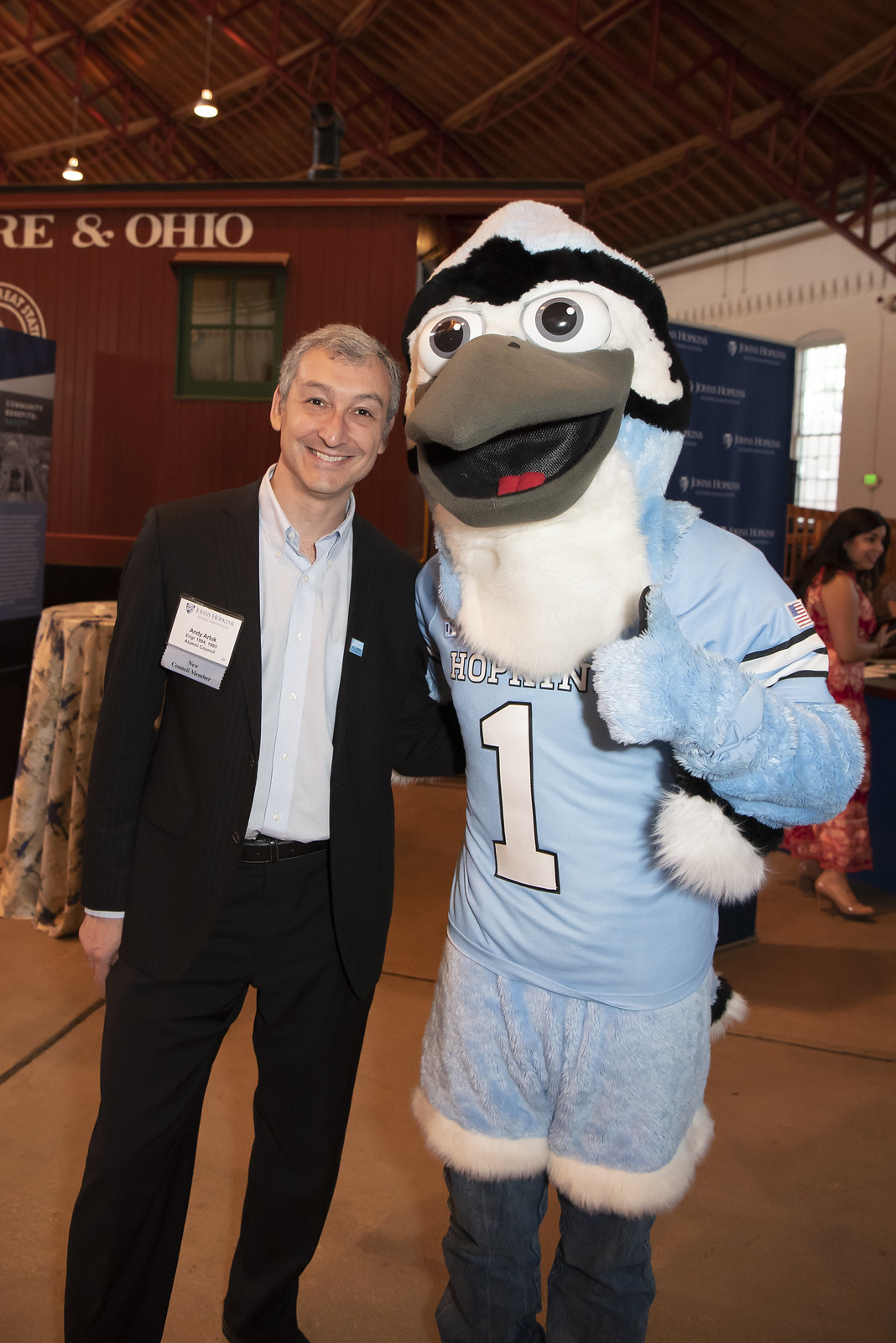In the image, we see a man named Andy Artuk, identified by his name tag that also labels him as a new council member at John Hopkins, standing next to a Blue Jay mascot. The Blue Jay mascot is dressed in a light blue outfit with a number one jersey, featuring distinct facial details such as white eyes with grey and black circles, a grey beak with a black interior and a red tongue, and black markings around the eyes. The mascot is also sporting blue shorts over blue jeans and is giving a thumbs-up gesture, with its arm around Andy.

Andy is wearing a dark suit jacket with no tie, complemented by a light blue dress shirt beneath. He has receding black and grey hair and dark eyes. Behind Andy and the mascot, the setting includes multiple people partially visible to the right and left, a maroon wood-paneled caboose with a green window, and part of a sign that appears to say "and Ohio." There's also a blue sign or divider panel and a white wall further in the background. Additionally, a small table is partially visible behind Andy, covered with a cloth. The enclosure they are in has an exposed wood beam ceiling and a cement floor, suggesting a semi-industrial or rustic indoor setting.